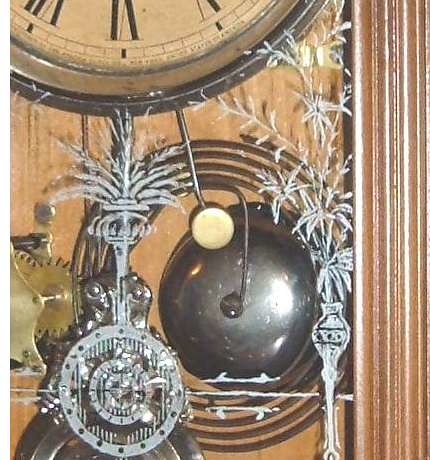This is an up-close color photograph of the intricate bottom half of a grandfather clock. The clock, encased in light brown wood, features a silver bell-shaped chime visible to the bottom left, likely used to strike the hour. The central focus is the large metal pendulum, adorned with floral or Victorian designs near its top and swinging beneath the round clock face. The clock face, partially visible, has a black border with a lighter beige background, and black Roman numerals.

A protective glass cover, etched with ornate designs, shields the pendulum and clock mechanism. The glass features detailed white etchings; one resembles a tall vase with leaves and flowers, positioned more to the left of the image, while another mimics a pocket watch with a long stem situated to the right. An intricate wire runs from the pendulum through the top, looping around the silver bell four to five times. The combination of these details with the wooden encasement and precise engravings showcases the timeless craftsmanship of the clock.